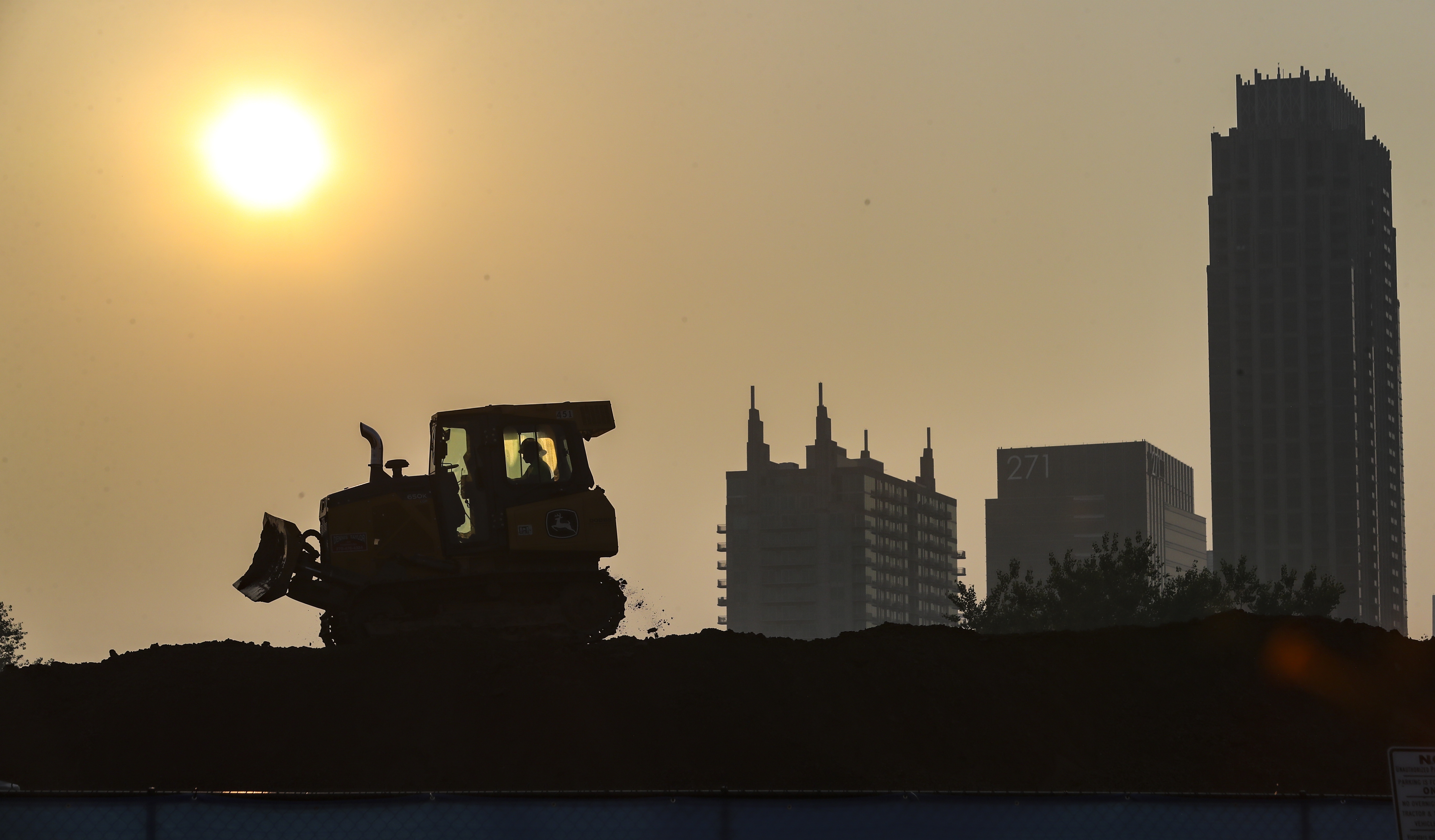In this landscape photograph, taken during the evening as the sun is setting, the sky is a hazy gray with a bright, blurred yellow sun positioned in the upper left-hand corner, casting a faint illumination across the scene. On the top left, there's a silhouette of a tractor-like construction vehicle with its shovel raised, heading leftward on a dirt pile. The lower portion of the image, stretching from the bottom left to the bottom right, is enshrouded in darkness, almost black, with mounds of dirt and small patches of green grass barely visible. In the background, on the right side, three buildings are outlined against the darkening sky: the closest one resembles an apartment building with approximately seven to eight floors, followed by a slightly smaller structure, and further to the right, a prominent high-rise skyscraper. A small bush is also noticeable on the left side near the dirt pile.